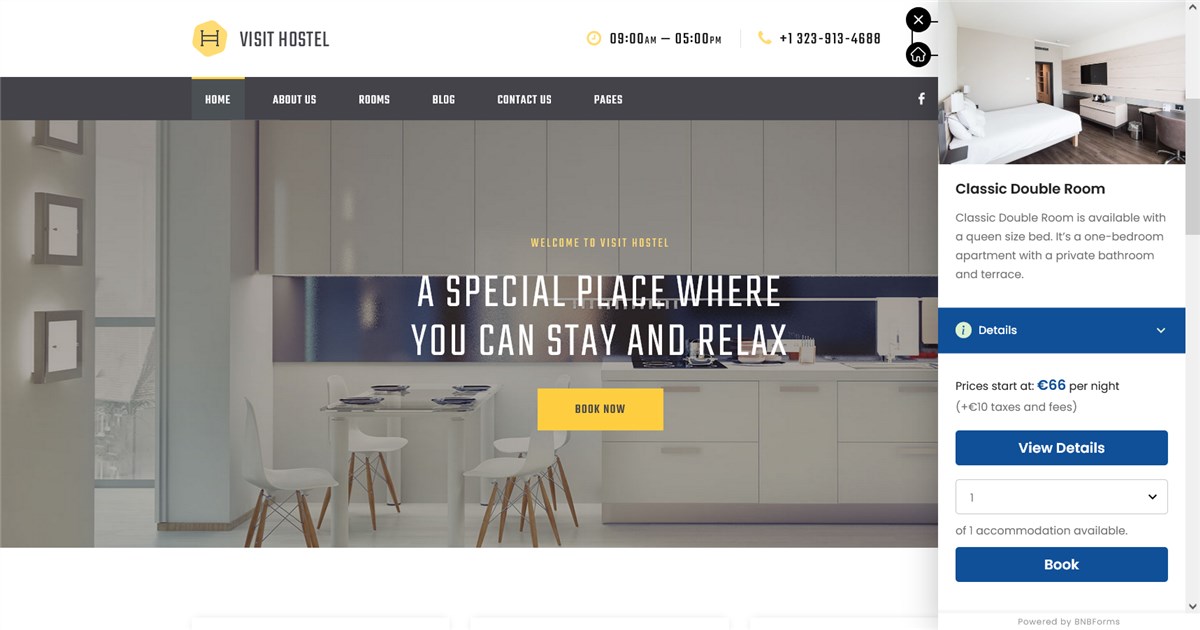The webpage depicted is a website for booking hostel accommodations named "Visit Hostel." In the top left corner, the site prominently displays its name alongside a distinctive yellow logo featuring a chair. Adjacent to this, the website indicates business hours, "9 a.m. to 5 p.m.", followed by a contact phone number: (132) 391-3468.

Occupying the upper portion of the page is a comprehensive navigation bar, facilitated by dark, earthy tones that provide a sophisticated backdrop. This navigation menu includes links to Home, About Us, Rooms, Blog, Contact Us, and Pages, with the Home button currently highlighted.

The central section of the homepage showcases a contemporary kitchen setting characterized by sleek, modern aesthetics. The kitchen is furnished with pristine white cabinets, white furniture, white kitchen chairs, a glass-topped table, and a white countertop. This ensemble is complemented by white drawers, creating a cohesive and modern look. Above this image, the welcoming message "Welcome to Visit Hostel" introduces the site as "a special place where you can stay and relax." Beneath this welcoming message, a prominent yellow button invites visitors to "Book Now."

On the right side of the page, a visual display of a classic double room is featured. This room includes a large, white bed, resembling a hotel room but catered to hostel standards. This descriptive visual presentation aims to attract potential guests looking for a comfortable and stylish place to stay.